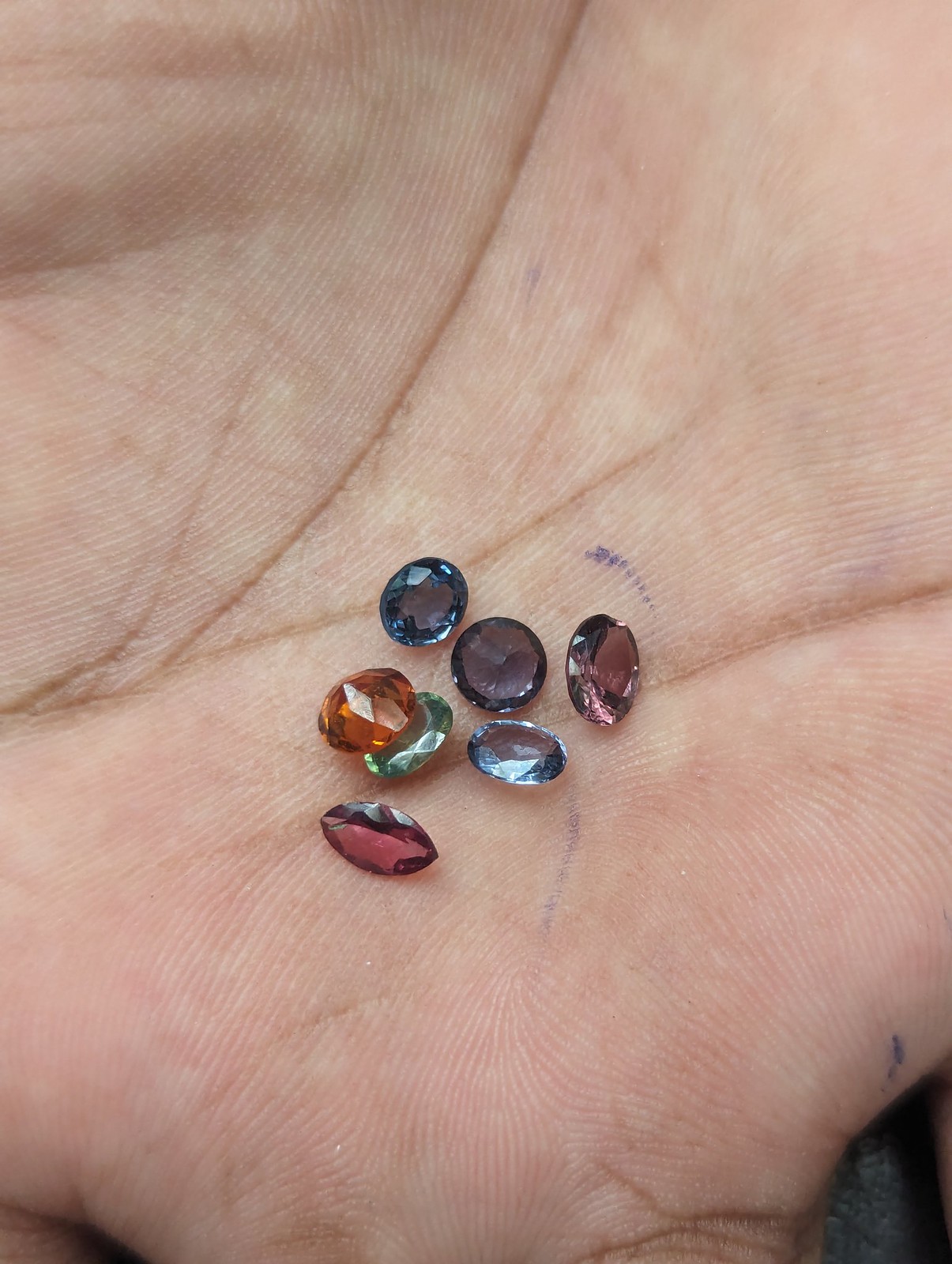The image is a close-up of a dirty, ink-marked human palm, where seven intricately cut precious stones rest haphazardly. The zoomed-in shot highlights the swirls of fingerprints and deep creases of the palm, which are filled with dirt. Several smudges of blue ink from a pen are visible on the hand, scattered around the gems. The stones exhibit a variety of vibrant colors, including different shades of blue, from dark to light, as well as orange, red, green, and purple. Their small size and the precise cuts enhance their multi-faceted appearance. Despite their varied positions—some lying flat, others standing on their edges—they are all clustered in the center of the hand.